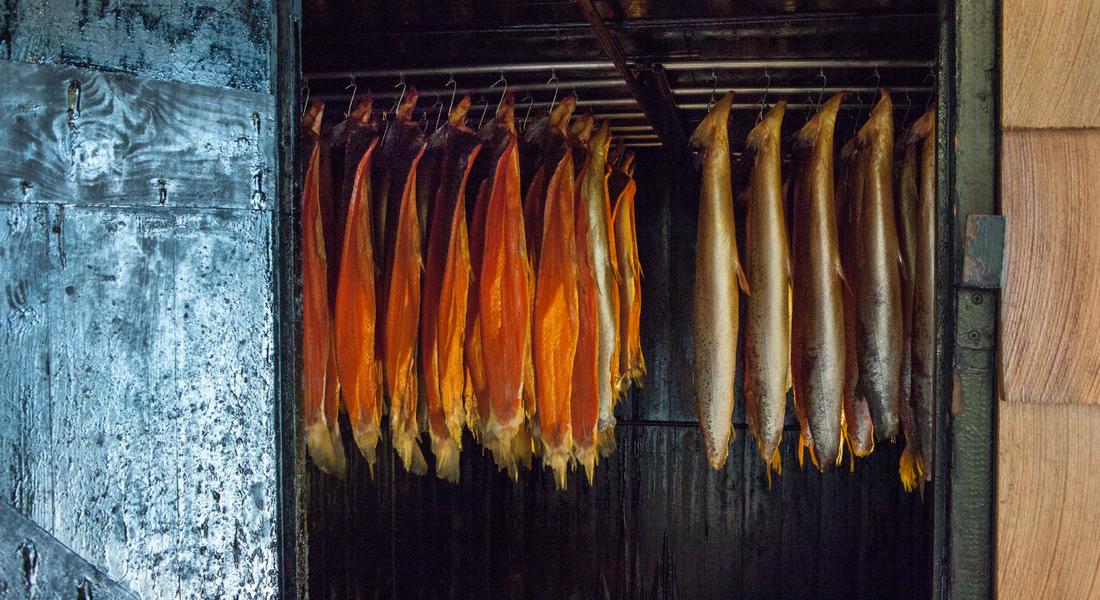This image depicts the interior of a dilapidated shed-like building constructed from worn-down metal and wood with a predominantly brown, blue, and steel-colored exterior. The photograph is taken from an open door that provides a view inside, revealing a rustic and grungy atmosphere. The ceiling features approximately seven metal rods from which numerous fish are suspended by hooks. On the left side of the room, there are vibrant orange-hued fish hanging in rows, while on the right side, there are more subdued grayish or tan-colored fish, with at least five visible rows extending into the darkened depths of the room. The shed's interior is shadowy, with wooden and metal elements making up its structure, and the roof appears particularly grungy with rust patches and darkened wooden walls in the background. Bright orange fish contrast with the somber tones of the environment, suggesting the fish are in the process of drying or being stored. The overall scene captures a sense of neglect and decay, highlighted by the rusty, old silver door and the weathered building materials.